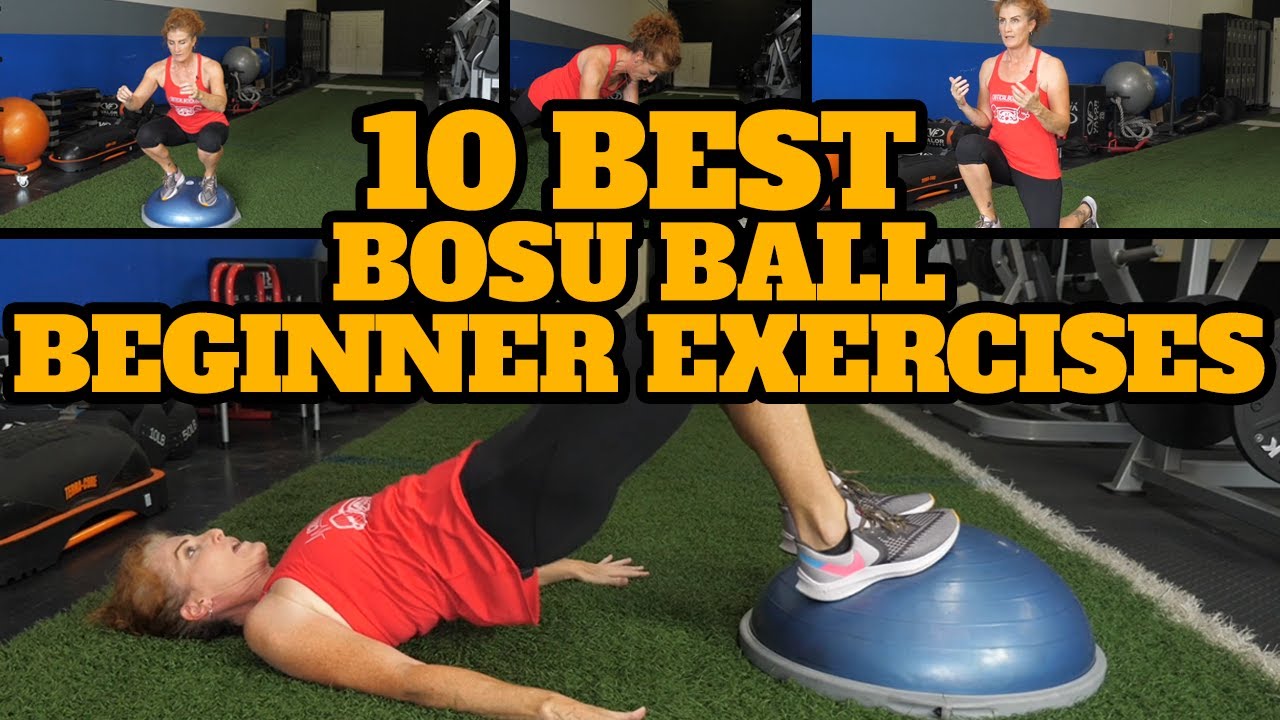The image is a YouTube thumbnail promoting "10 Best BOSU Ball Beginner Exercises." It features a vibrant orange title with a black outline prominently displayed over a collage of four different photographs. The host of the video, a young woman clad in a red tank top, black leggings, and Nike sneakers, demonstrates various exercises using a BOSU ball in each photo. The top left image shows her squatting on the BOSU ball, showcasing balance and strength. The middle left image, slightly obscured by text, likely depicts her performing push-ups with her hands on the BOSU ball. The top right image shows her in a lunging position, emphasizing stability and form. The large bottom image captures her in a hip thrust position, with her feet on the BOSU ball and her shoulders on the ground, lifting her hips upward. The BOSU ball itself is a half-ball with a stable platform, used for versatile, effective workouts.